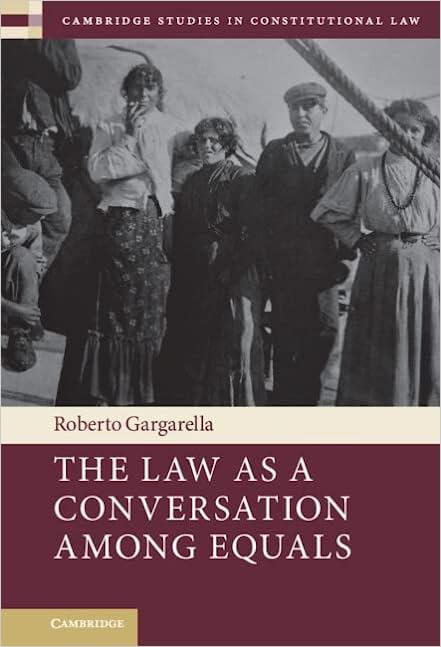This poster showcases a historical photograph likely set during a wartime period in a distressed zone. Prominently featured on the left are two women with short hair. The taller woman, dressed in a white blouse and long skirt, appears to be smoking a cigarette. Beside her stands a shorter woman in dark-colored clothes, including a cap, with a long-sleeve dress. There are also a few men partially visible on the far left, their heads or parts of their bodies cut off by the photograph's edge. Another woman, somewhat obscured by a rope in the upper left corner, wears a black necklace, a long-sleeve top, and a long skirt.

At the top of the poster, in maroon, reads "Cambridge Studies in Constitutional Law." Beneath the photograph, it lists the author "Roberto Gurella" on the left. Below this, also on a maroon background with white lettering, the title "Law as a Conversation Among Equals" is prominently displayed. The lower left side of the poster features the word "Cambridge" repeated in white font against a gold background, highlighting the affiliation with Cambridge University.